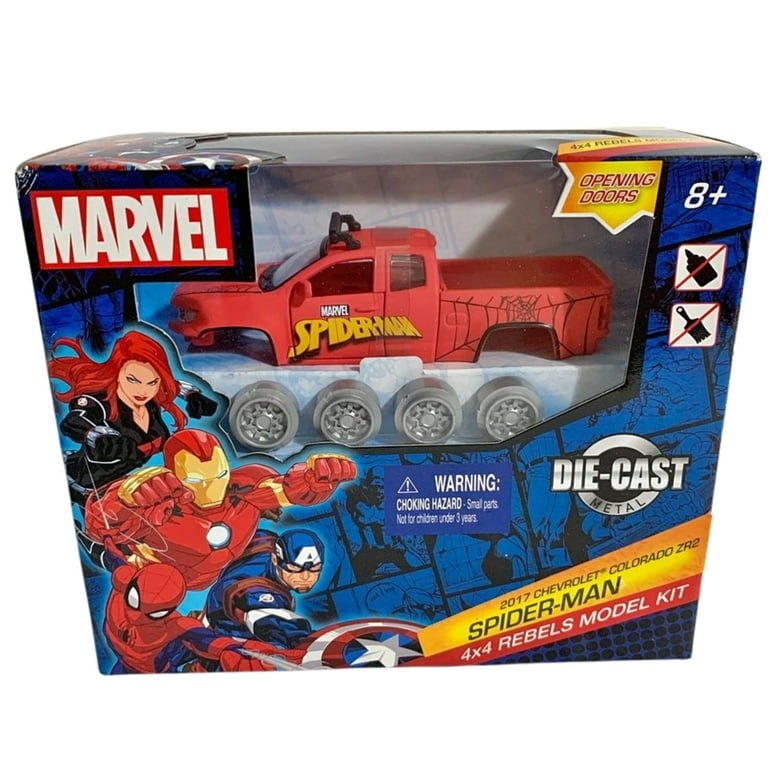This toy product features a detailed box design with blue, comic book-style art showcasing various Marvel characters in action panels. Prominently displayed in the upper left corner is the traditional Marvel logo, written in white font on a red block. The upper right corner of the box highlights the age recommendation, "8+", along with a yellow starburst pattern stating "Opening Doors." The product itself is a model kit for a 2017 Chevrolet Colorado ZR2 Spider-Man 4x4 Rebels pickup truck, depicted in red with intricate details such as a spider web on the truck bed and "Marvel Spider-Man" on the driver's side door. It includes four sets of silver rims, a black light on top, and die-cast metal components, which do not require painting or gluing. The front of the box features a clear cutaway window to view the truck and rims. On the left side of the box, an array of Marvel superheroes—Black Widow, Iron Man, Spider-Man, and Captain America—are illustrated in vibrant detail. Safety information, including a warning about small parts being a choking hazard for children under 3, is also prominently displayed, alongside icons indicating no need for glue or paint.